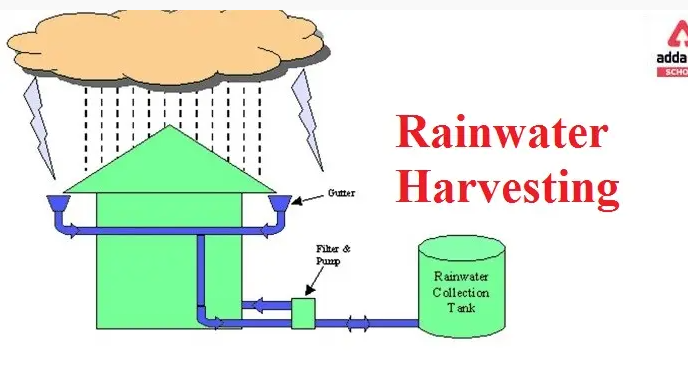The illustration depicts the steps involved in rainwater harvesting with vivid details and clear labels. On the right side of the image, "Rainwater Harvesting" is prominently displayed in red text. The diagram begins with a light orange cloud on the left, featuring lavender lightning bolts and dotted lines to indicate rain. The rain falls onto a green house with a pyramid-shaped roof that channels the water into blue gutters labeled "gutter" in black text. These gutters direct the water to a green box marked "filter and pump." Arrows indicate the flow, with the water finally ending up in a labeled, circular rainwater collection tank. The visual elements include the cloud, house, gutters, filter and pump box, and the collection tank, making the process of harvesting rainwater easy to understand.